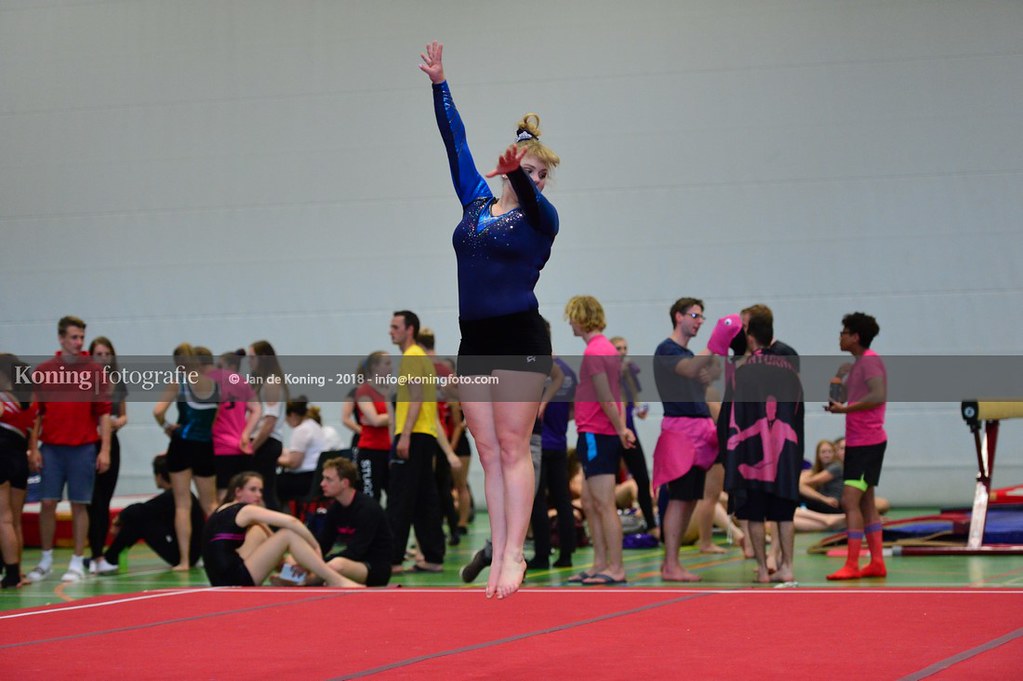In this image, a gymnast is captured mid-pose on a red floor mat, her body elegantly straight with both feet off the ground. She is wearing a blue sequined top with black stripes and black shorts. Her blonde hair is styled in a bun, and she raises her arms above her head while looking towards her left. In the background, a large white cinder block wall extends across the upper half of the image, featuring a light gray rectangular banner in the center with the text "Koning Photography Jan de Koning - 2018 info@koningphoto.com" in white font.

The scene appears to be set in a gymnasium, with a green gym floor adjacent to the red mat. Various individuals are present in the background, dressed in sports attire. Some appear to be competitors in pink outfits, while others, possibly coaches, wear casual attire such as a man in a red sweatshirt and blue jean shorts. They are either standing, talking, or preparing for what seems to be a competition or gymnastics event.